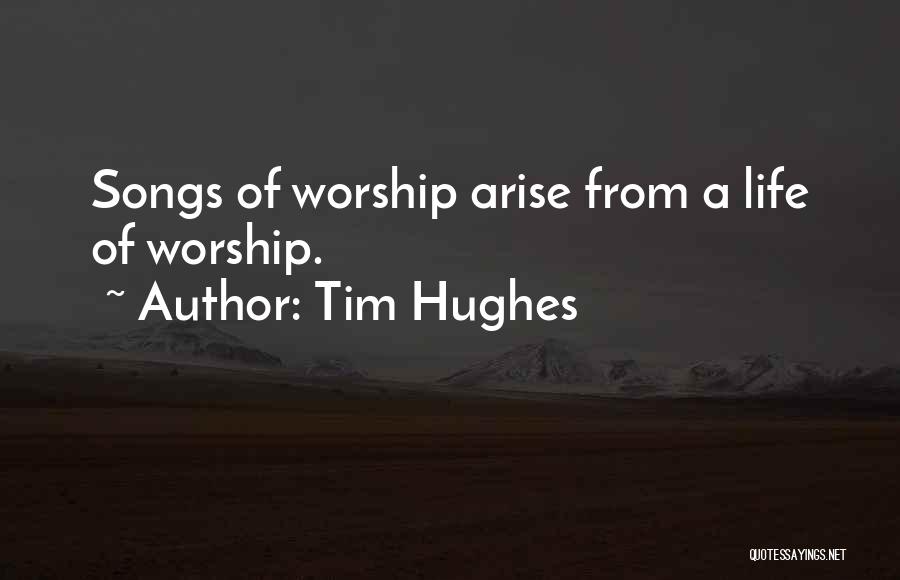In this dark, nighttime photograph, a vast landscape is depicted, showcasing a large plot of mostly dirt and a few scattered trees in the foreground. Greenery peeks through behind the rugged earth, leading the eye towards the majestic, snow-capped mountains that rise prominently in the background. The scene suggests a locale reminiscent of Colorado, Utah, or Wyoming, where expansive flatlands meet towering peaks.

White text stands out sharply against the darkened scenery, reading, "Songs of Worship Arise from a Life of Worship," attributed to Tim Hughes. This stark contrast draws the viewer's attention immediately to the inspirational quote. Additional text, "QuoteSayings.net," subtly appears in the bottom right corner, indicating the source of the quote.